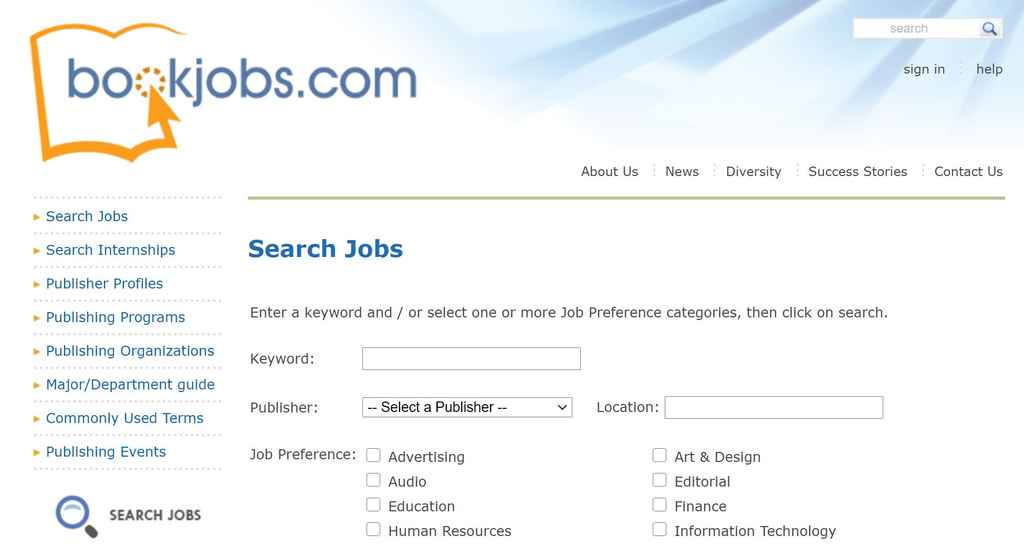Here's a detailed and descriptive caption for the image:

"An extensive selection of resources and tools available at Jobs.com, aimed at bringing diverse job opportunities to aspiring professionals in the publishing industry. Featuring intuitive search functionalities, including keyword, publisher, and location filters, the platform caters to a variety of job preferences such as Advertising, Audio Education, Human Resources, Art and Design, Editorial, Finance, and Information Technology. Beyond job searches, Jobs.com offers comprehensive guides and information on major departments, publishing terms, events, and success stories. Discover more about us, our commitment to diversity, and how we can help you succeed by visiting https://www.jobs.com."